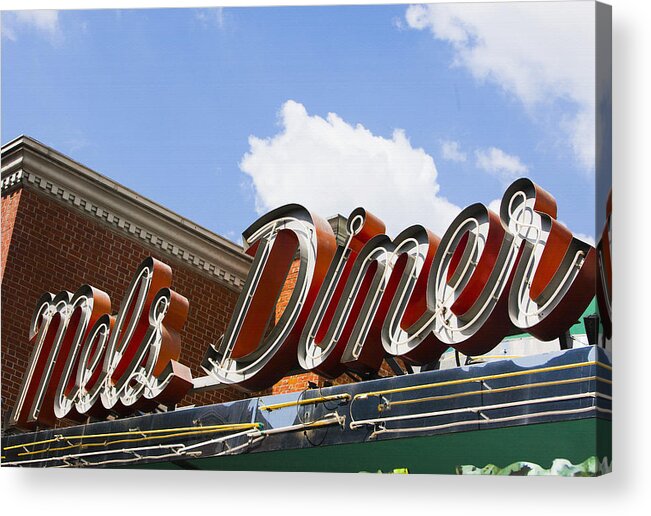The image showcases a canvas art piece featuring the iconic signage of "Mel's Diner." The focal point is the vivid neon sign, which prominently displays "MEL'S" in italicized, casual writing with white neon tubing. Below "MEL'S," the word "DINER" is stylized similarly in neon, adding to the retro charm. The sign is bordered in red, creating a striking contrast against the blue sky adorned with white clouds.

To the left of the sign, there's a brick building with distinctive designs at the top of its flat roof, adding architectural interest. The facade of the diner itself features a purple-gray backing at the top, accented with additional neon tubing in white and yellow that run horizontally to add vibrant color. Below this, the front of the building is finished with green material, framing the entrance and giving the diner its unique look. The blue roof edge further accentuates the colorful aesthetic of this memorable diner scene, all captured on a canvas-style artwork.